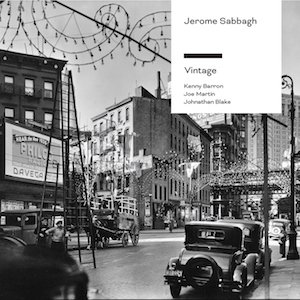This black-and-white photograph captures a bustling city street scene, likely from the late 1910s to the mid-1930s, notable for its period details. Dominating the image are several multi-story commercial buildings, including a large brick structure on the left side. Prominently visible is a billboard on the left-hand side that reads "Philco." Vintage cars, reminiscent of the Model T era around 1925, are parked along the streets, and there is even a horse-drawn buggy amidst them. A peculiar element in the image is a giant ladder situated in the middle of the street. Streetlights with decorative scrollwork add to the period charm. In the upper right corner of the image, a white rectangular sign with black lettering reads "Jerome Saba," followed by a black horizontal line under which words like "Vintage" and names such as Kevin Barron, Joe Martin, and Jonathan Blake are inscribed. The street is abuzz with people going about their day, capturing the essence of an early 20th-century urban landscape.